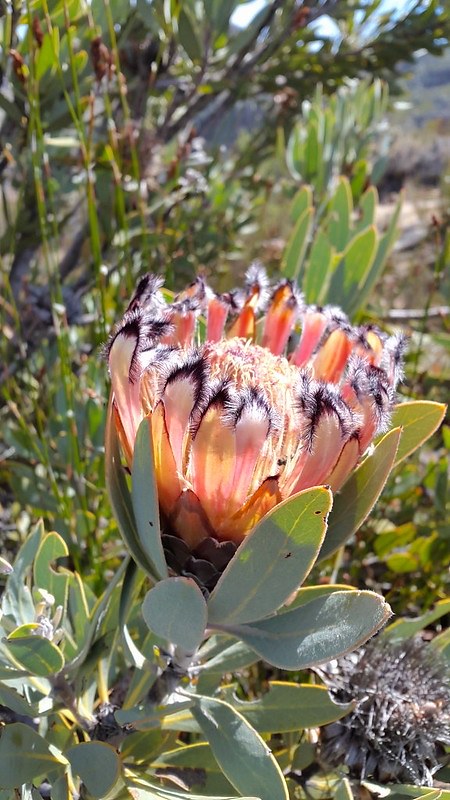The photograph captures a vibrant outdoor garden scene featuring a striking and elaborate plant with a large, eye-catching flower. The flower stands out with a dramatic array of petals, numbering between 10 and 20, that encircle its core. The petals are a medley of colors, featuring shades of pink, red, orange, and white, with distinct black tips and a delicate white frill at the ends, resembling bird feathers. The flower's intricate design hints at a potentially carnivorous nature, with furry spines and a claw-like arrangement that could suggest a bug-eating capability. The plant itself boasts long, slender green leaves that shoot up from a robust stalk. Surrounding this captivating flower are numerous other plants, including skinnier stalks and a nearby tree, contributing to the lush greenery of the garden area.